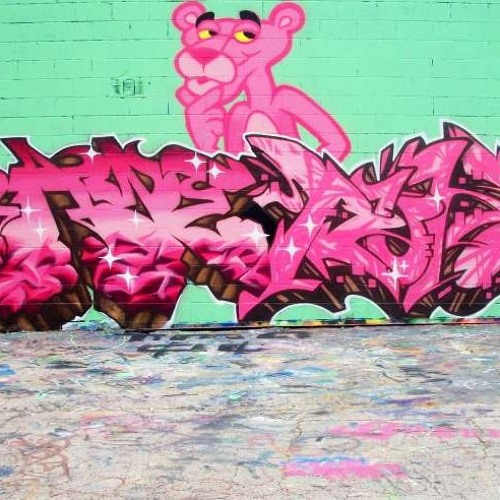The image depicts a vivid, lime green brick wall covered with a striking mural of the Pink Panther. The Pink Panther, instantly recognizable with his sleek, pink fur, yellow eyes, and thick black eyebrows, strikes a contemplative pose with his chin resting on his right hand and his eyes gazing thoughtfully upward. His left arm is visible down to the elbow, and his light pink chest contrasts with his darker pink nose and mouth. Below him, intricately painted graffiti adds an additional layer of artistry to the wall, featuring shades of pink and purple with brown accents and white stars scattered throughout. The graffiti includes letters with varying shades of pink and intricate shading, although they are not easily readable. The floor in front of the wall, likely a concrete sidewalk, is splattered with colorful bursts of spray paint, complementing the vibrant mural. The mural spans the height of the wall, merging street art with the iconic imagery of the Pink Panther.